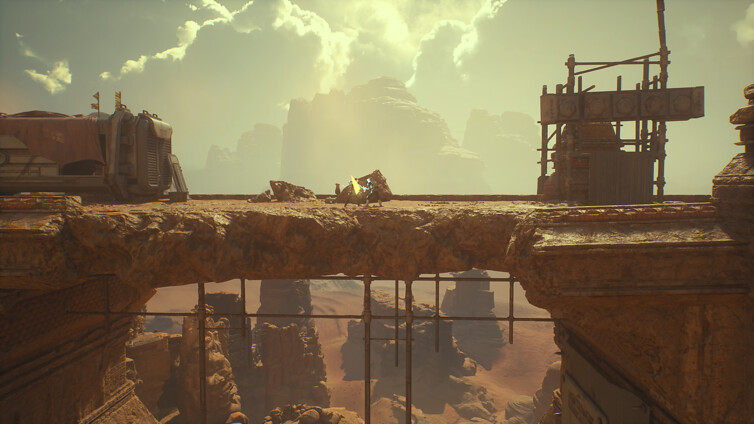In this intricate computer-generated image, a brown bridge spans a vast desert scene scattered with numerous rock outcroppings. The bridge, appearing prominently in the foreground, houses several buildings and features a transportation vessel positioned on the left side. On the right side of the bridge, a framework or structure is seen, seemingly in the process of constructing or holding an egg-shaped object. At the center of the image, two men, depicted very small, are engaged in a fierce battle involving fire, situated on the bridge or archway that offers a view of the desert below through an opening. Dominating the background, large gray cumulus clouds loom over the scene, with smoggy rock outcroppings faintly visible in the distance. The overall color palette is warm and earthy, with the bridge and background rendered in various shades of tans and browns, enhancing the sense of heat enveloping the landscape.